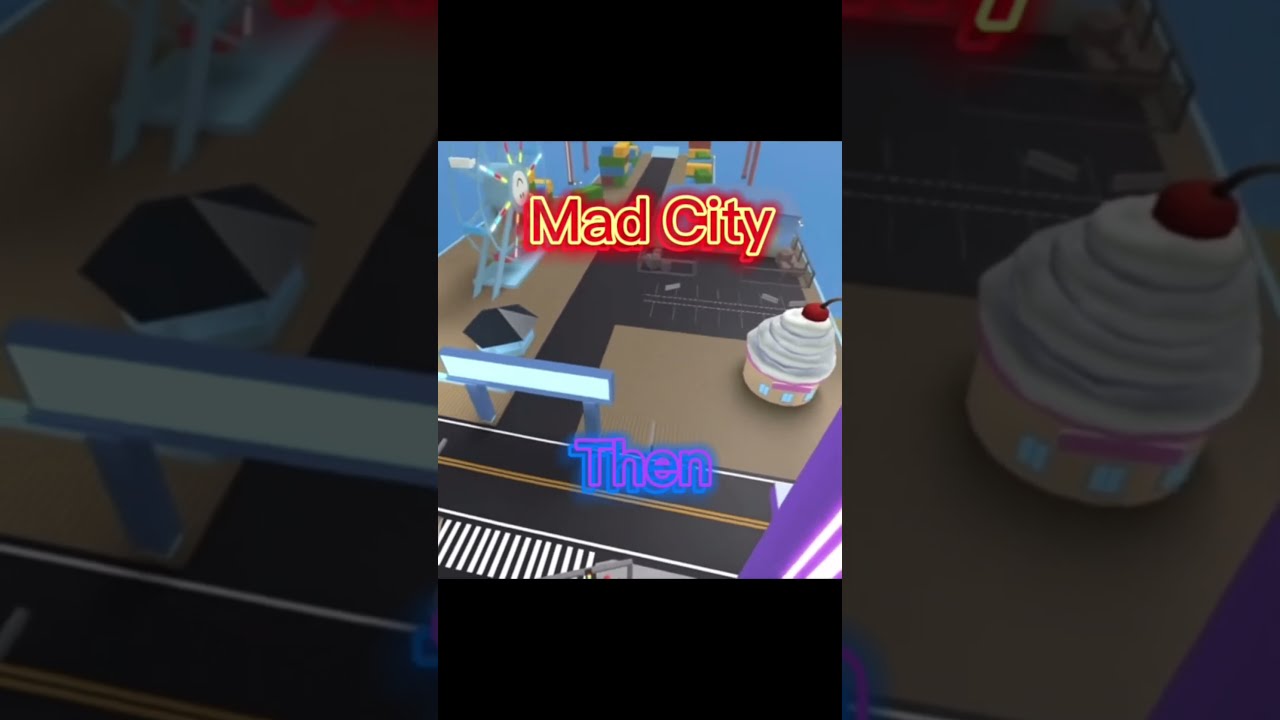The image showcases a vibrantly designed artwork that appears to be for a game titled "Mad City," with the title prominently displayed in glowing red and yellow letters at the top. Below, the name "Ben" is written in purple and blue letters with a similar glow effect. The central scene is framed within a square against a darker, shadowed background of the same scene.

In the scene, a detailed street layout is depicted, featuring a whimsical cupcake building with white cream and a cherry on top, situated on the right side. Opposite this cupcake building is a shop with white walls and a triangular black roof. In the background, a colorful Ferris wheel, resembling those found on an Atlantic City pier, stands out against a blue backdrop. Surrounding the Ferris wheel and street are vibrant green, yellow, blue, and red blocks reminiscent of a pixel or block-style game like Minecraft. The overall composition suggests an imaginative, game-like cityscape full of playful elements and bold colors.